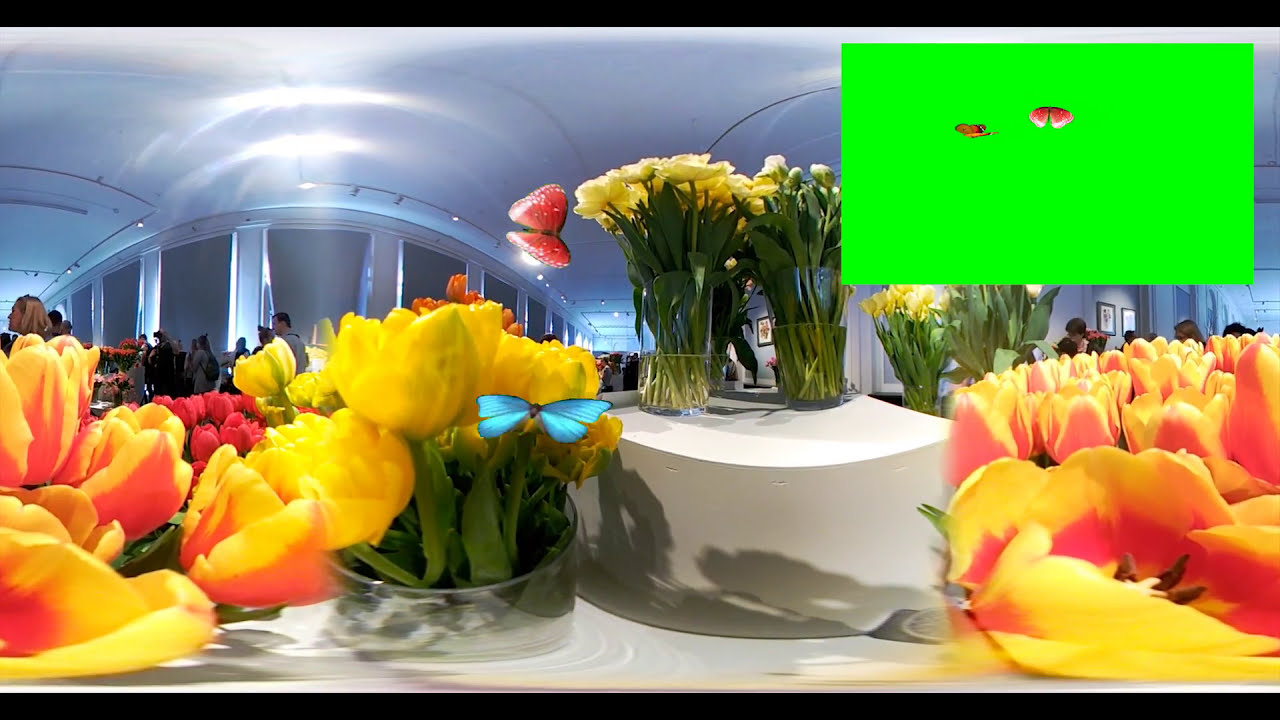The image depicts a large, indoor conference hall filled with clusters of yellow, pink, and mixed tulips arranged in clear glass vases. A prominent pink butterfly floats above the tulips just left of center, with other red and light blue butterflies also edited onto the flowers. In the background, several people are standing and seated, engaged with something off to the left and towards the center of the room. The room features a light gray color scheme and has portraits or pictures mounted on the walls. In the upper right corner, there is a solid lime green rectangle with a small depiction of a chrysalis and a butterfly, adding an additional layer of visual interest to the scene.